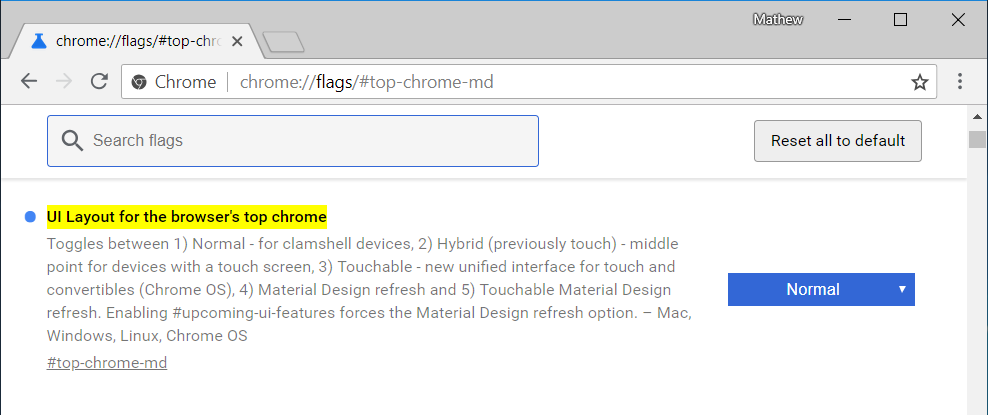In this image, we are presented with a screenshot of a Chrome browser window focused on the experimental features page, identifiable by the URL "chrome://flags/#top-chrome-md" displayed in the address bar. The top section of the window is a light gray color bordered with blue and black accents. Below, a search box within a gray container is prominently visible, labeled "Search flags," accompanied by an option to "Reset all to default" on the right side.

In the upper-right corner of the screen, "Matthew" is displayed in white text, indicating the logged-in user’s profile. Central to the image is a section with a blue bullet point next to a detailed description of the UI layout options for the browser's top chrome. The description enumerates five toggle options: 

1. Normal, designed for clamshell devices.
2. Hybrid, previously known as touch.
3. Touchable, a new unified interface for touch and convertible devices.
4. Material Design Refresh.
5. Touchable Material Design Refresh, which enables upcoming UI features.

These options are noted to be compatible across multiple operating systems including Mac, Windows, Linux, and Chrome OS.